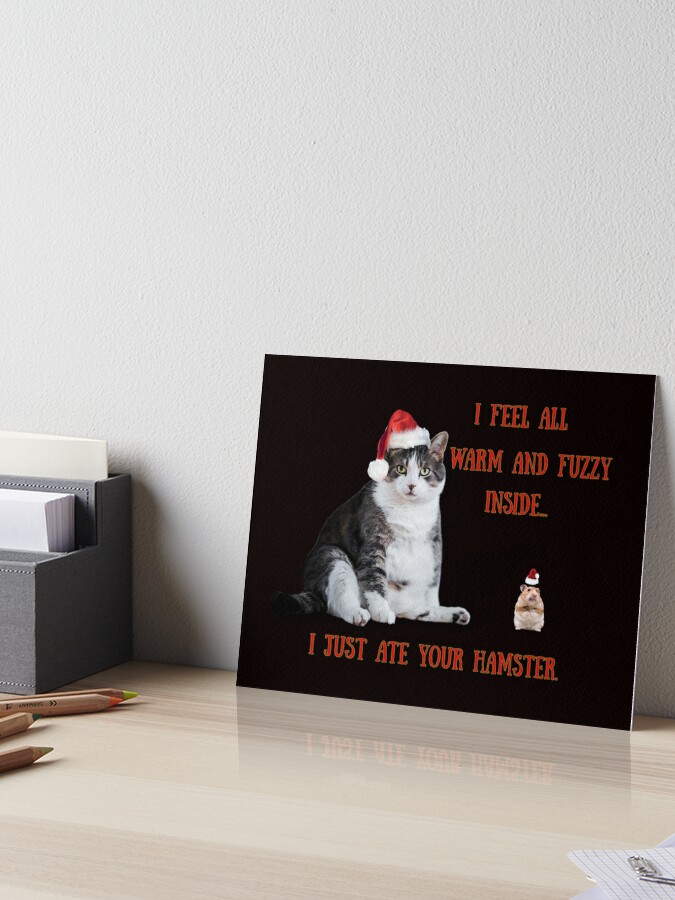In the image, a humorous sign is propped against a white wall, situated on a glossy, pale wooden table. The sign itself is black with red text at the top that reads "I feel all warm and fuzzy inside" and below that, "I just ate your hamster". The sign features a whimsical illustration of a large, plump cat with white and black fur, seated in the left half of the sign area, wearing a Santa Claus hat. To the right of the cat is a small tan hamster, also donning a Santa Claus hat. Both characters face forward, creating a comical scene.

In the lower right corner of the image, partially visible, are some notebook ruled papers and paper clips. To the left, a gray index card holder or envelope container is visible, holding several envelopes. In front of this holder, four colored pencils, in shades of yellow, orange, green, and possibly white, are scattered on the table, adding a touch of color to the scene. The whole setup conveys a playful and slightly mischievous holiday vibe.